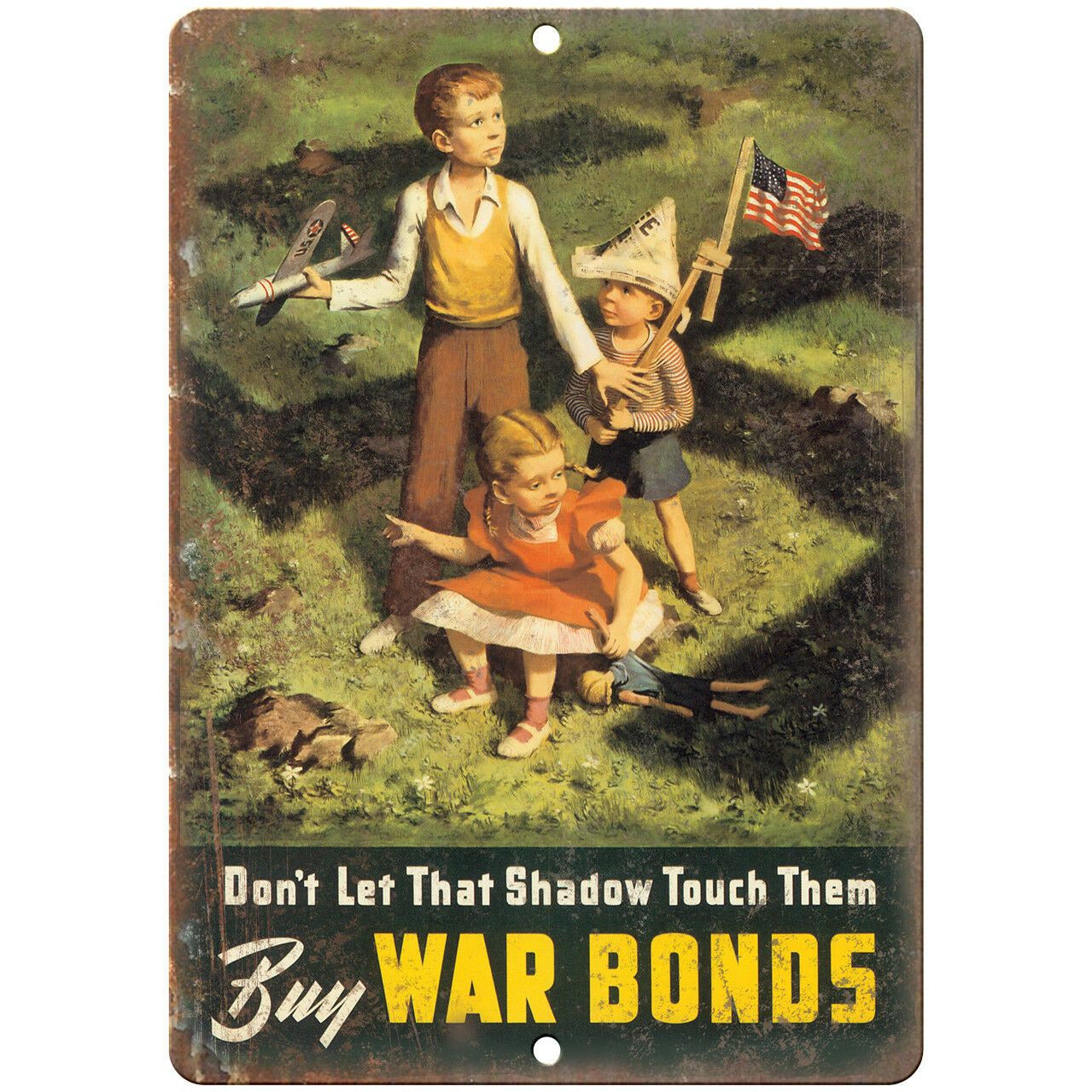This detailed wartime illustration, used as a World War II War Bonds advertisement, features a powerful scene of three American children standing in a grassy field. The backdrop is dominated by the menacing shadow of a Nazi swastika, symbolizing the threat of war. In the foreground, an older boy, dressed in a yellow collared long-sleeved shirt with a white collar and brown pants, clutches a gray U.S. airplane marked with a star in his right hand. Adjacent to him, a younger boy wearing a red and white striped shirt and blue shorts, sports a newspaper hat and holds an American flag taped to a wooden board. In front, a little girl with blonde pigtails, adorned in a red dress with a white pinafore, sits on the ground holding a doll that mirrors her appearance, complete with a blue shirt and black pencil skirt. Both boys wear white sneakers with red socks. The grassy field they stand on is dotted with small white flowers and rocks. Above them, the foreboding message reads, "Don't let that shadow touch them," in white letters, followed by "War Bonds" in yellow font, urging viewers to support the war effort.